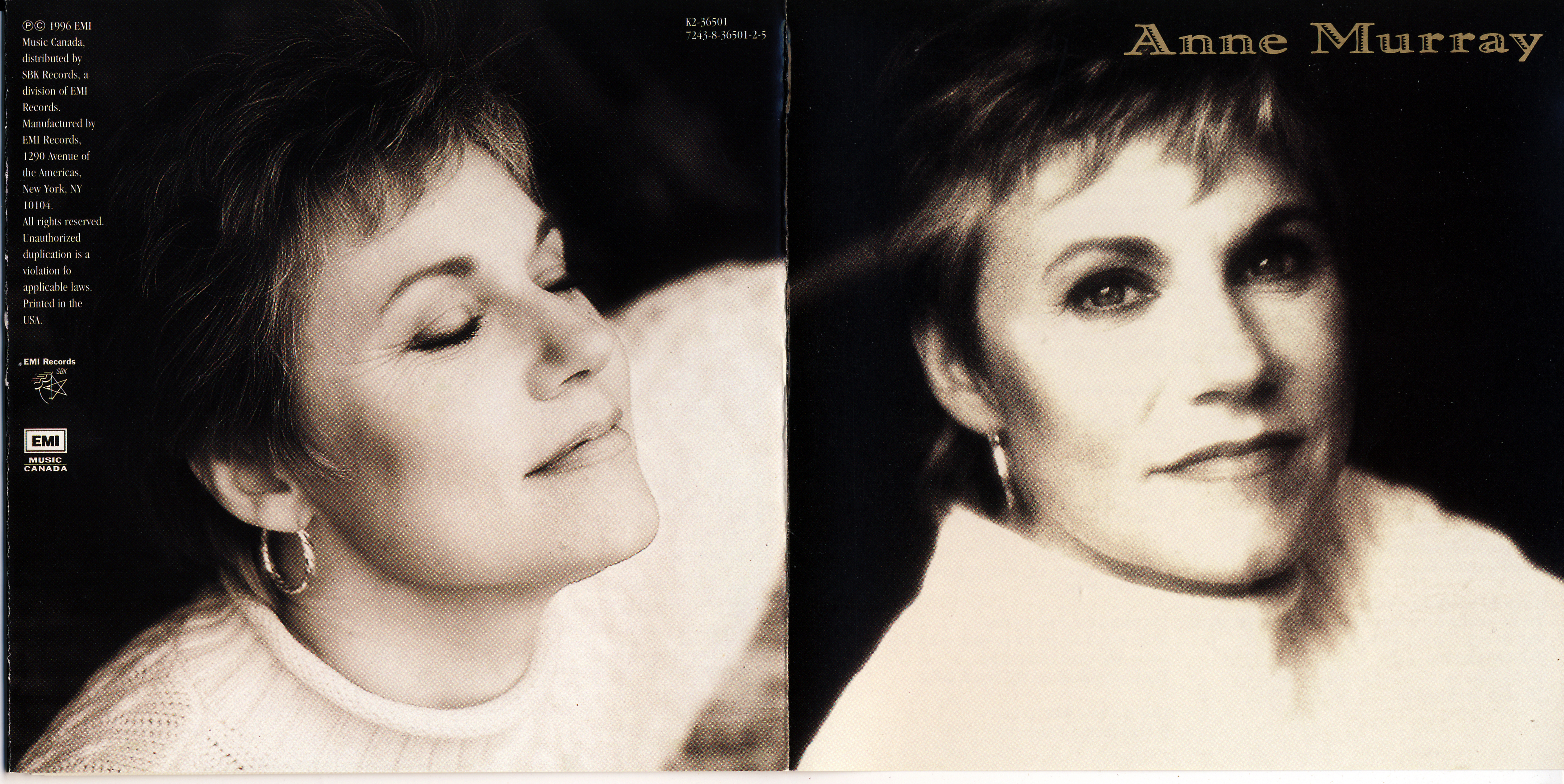The album cover image features two side-by-side black-and-white photos of the same woman, showcasing both the front and back of the album. The woman is wearing a long white sweater and has short, blondish-tipped hair. She is adorned with earrings and makeup. 

In the left image, which represents the back cover, the woman is seen with a gentle smile, eyes closed, and her face turned slightly upward towards the sky. There are texts on both the top left and the top right corners of this left image, though the words are small and difficult to decipher. Notably, it mentions EMI Records and EMI Music Canada.

In the right image, signifying the front cover, the woman looks directly at the camera with her eyes open, displaying a similar gentle smile. The text at the top right of this image reads "Anne Murray." The overall setting of the photos is enhanced by clear lighting, aiding the visibility of details in the black-and-white and beige-toned images. On the back of the album, a list of all the songs is also provided.